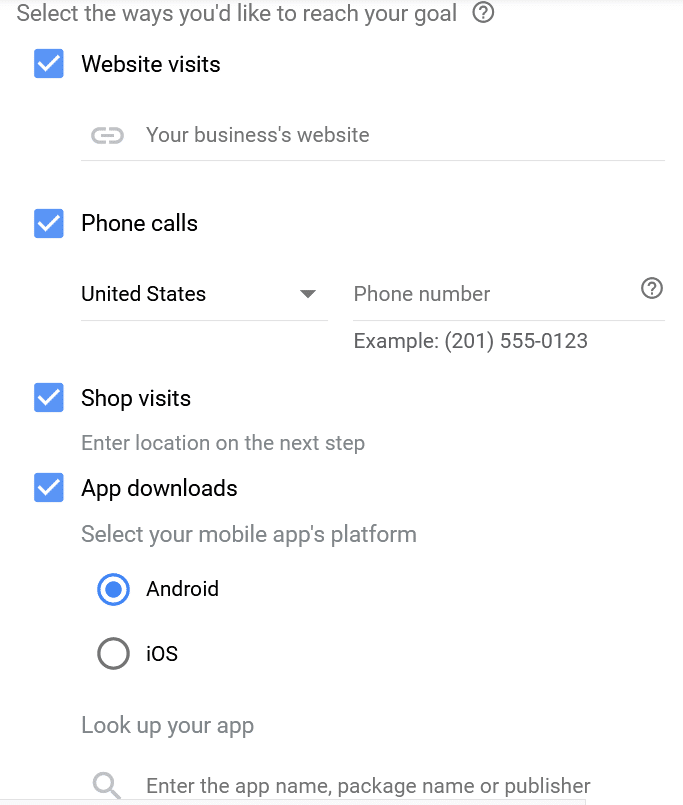A detailed control panel interface for managing goal achievements is displayed. At the top, bold text reads "Visit Websites," suggesting this section involves directing users to various online destinations. Adjacent to this is an instruction: "Select the ways you'd like to reach your goal," followed by a gray circle containing a question mark, indicating the availability of additional help or information.

Below this header are four main options, each implemented with blue checkboxes containing white check marks, signifying that all options are currently active.

1. **Visit Websites**: This section includes a link titled "your business's website," although the specific URL or destination is not provided.
   
2. **Phone Calls**: This part features a drop-down menu set to "United States" and a sample phone number formatted as "201-555-0123," indicating where phone call tracking or interactions will occur.

3. **Shop Visits**: Instructions prompt the user to "enter location on the next step," suggesting that physical store visits will be tracked or targeted next.

4. **App Downloads**: Here, users are to "select your mobile app's platform," with "Android" already selected and highlighted in blue. An additional sub-option allows for app identification with an input field labeled "enter the app name, package name, or publisher," accompanied by a magnifying glass icon for searching.

Overall, this control panel appears designed to facilitate and monitor various user engagement strategies, such as website visits, phone contacts, physical store visits, and app downloads, presumably for marketing or analytical purposes. The intent is to track and enhance interactions leading to the achievement of specific goals.